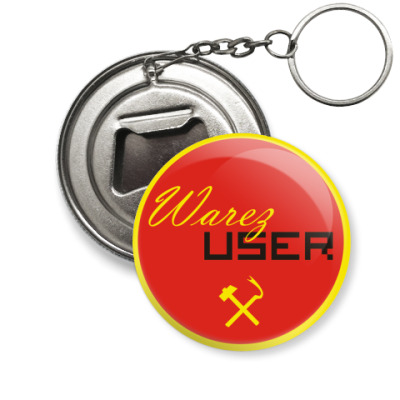The image features a silver keychain with a round red cover. The keychain consists of three linked silver rings culminating in a key loop, and it prominently displays both the front and back sides. The front side of the keychain, which is circular, showcases a narrow yellow band around its perimeter and a red center. Inscribed within the red circle, in yellow script, is the word "W-A-R-E-Z" overlaid by the word "USER" in black block letters. Below the text, there’s a yellow symbol resembling a crossed sledgehammer and crowbar. The back side of the keychain, which is entirely silver and metal, includes a functional bottle opener. The keychain is depicted with the red cover slightly offset to the bottom right, providing a clear view of both its detailed front design and practical back feature.